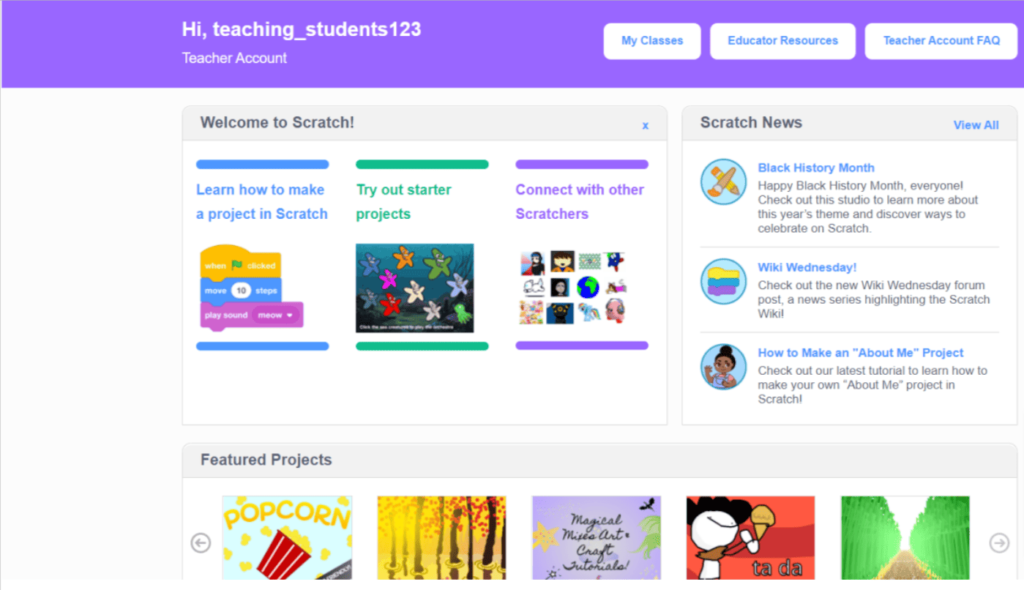On this educational website, the interface features a prominent purple bar at the top, displaying the greeting "Hi, Teaching_Students_123" in white text. Just below this, in a smaller white font, it identifies itself as a "Teacher Account." To the right of this bar are three buttons in white with blue text: "My Classes," "Educator Resources," and "Teacher Account FAQ."

Below the purple bar, the rest of the interface is set against a clean white background. There is a welcoming message within a box that reads, "Welcome to Scratch!" with three columns beneath it, each in different colors: blue, green, and purple. Each column offers different introductory activities. The blue column encourages visitors to "Learn how to make a project in Scratch" and features a small diagram with yellow, blue, and purple elements. The green column invites users to "Try out starter projects" and contains various colorful, star-shaped icons. The purple column prompts users to "Connect with other Scratchers" and includes multiple small icons. These columns are further separated by blue, green, and purple lines for clear differentiation.

On the right side of the page, there's a box labeled "Scratch News" with an option to "View All." The top news item highlights Black History Month, inviting users to explore the theme and find ways to celebrate on Scratch, with "Black History Month" highlighted in blue text. Below that, the "Wiki Wednesday" update, also in blue, encourages users to check out the new Wiki Wednesday forum post—a series focused on the Scratch wiki. Lastly, there's a tutorial on "How to make an About Me project," with the link in blue text guiding users to create their own personalized project. Small round icons accompany each news headline: a crossed pencil and paintbrush for Black History Month, a yellow, blue, and purple icon for Wiki Wednesday, and a cartoon of a little Black girl raising her arm for the "About Me" project tutorial.

Further down, a gray bar headlines the "Featured Projects" section, showcasing five different projects. The first project on the left is called "Popcorn," depicted with a popcorn box against a light black background, while the second project features a yellow background with black trees and foliage in yellow and red. The central project titled "Magical Mixes Art Craft Tutorials" stands out with its purple background. The fourth project showcases a person holding an ice cream cone with an excited "Ta-da!" set against a red background. The final project on the right depicts a scenic view with two rows of trees flanking a small road.